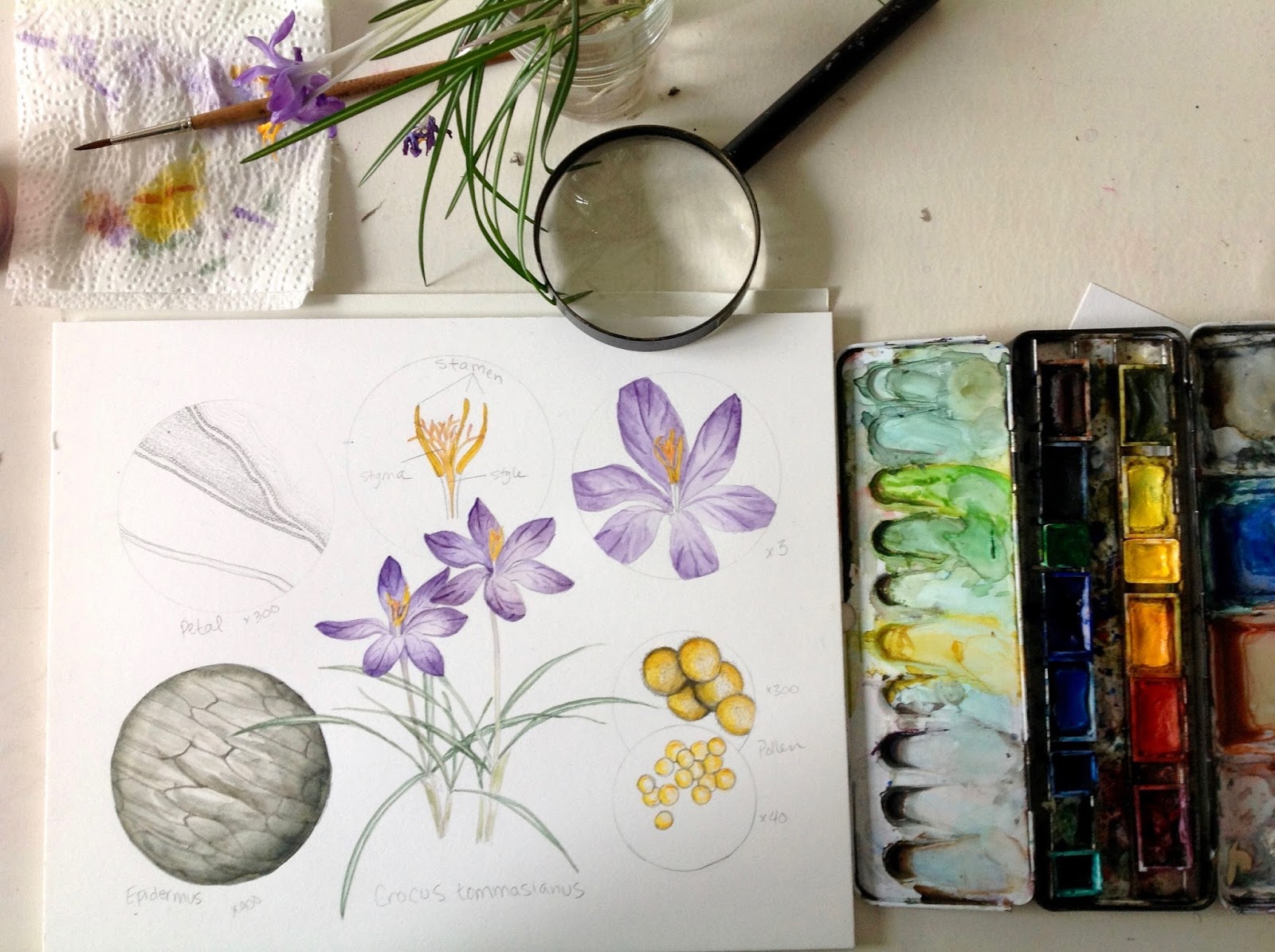The image captures an artist's workspace featuring a white canvas on a cream-colored desk. The canvas showcases detailed botanical illustrations of crocuses, including magnified views of the stamen, epidermis, petals, and pollen at various magnifications (3x, 45x, and 300x). These illustrations are painted with watercolors, with hues of purple, red, orange, yellow, black, white, blue, and green evident in the meticulous artwork. Adjacent to the canvas lies a heavily-used watercolor palette, complemented by a black magnifying glass positioned above the drawings. In the top left corner, a folded paper towel stained with yellow and purple paint marks is visible, indicating where the artist has cleaned their brush, which rests atop the towel. A small mason jar filled with real crocus flowers, submerged in water, is placed next to the canvas, mirroring the illustrations. The combination of detailed scientific artwork and vibrant live specimens creates a vivid portrayal of the artist's dedication and skill.